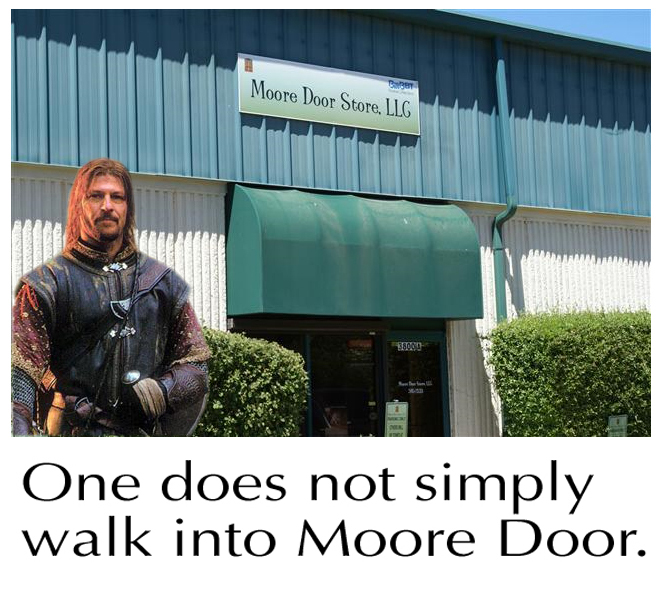The image is a meme featuring Sean Bean as Boromir from "The Lord of the Rings," standing to the left of a shopfront named "Mordor LLC." Boromir is depicted in his characteristic battle attire with long brown hair, a black vest, a red undershirt adorned with gold fringes, long gloves with mesh on the forearms, and a shield on his back. The shopfront above him features a sign with black text on a white background, placed on corrugated blue metal, that reads "Mordor LLC." Below is a green awning covering the doorway, which is framed by hedges on either side and set against a white lower exterior wall. The sky peeks through in the top right corner, revealing a bright blue, indicating a sunny day. Below the image, in bold black text on a white background, it reads, "One does not simply walk into Mordor."